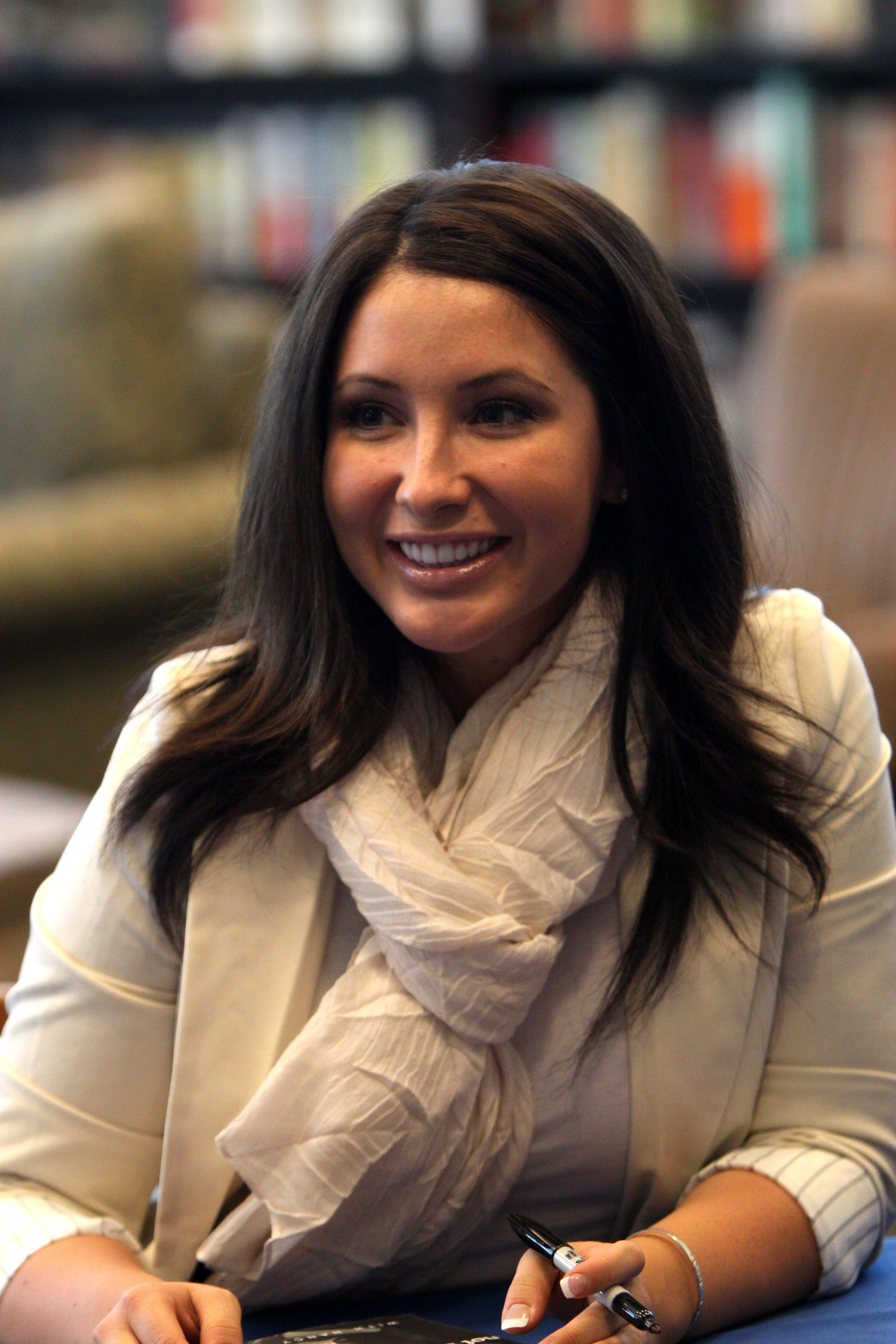In this indoor daytime scene set in a library, we see a young woman positioned centrally in the image. She is seated at a table draped with a blue tablecloth, surrounded by blurred bookshelves and lounge chairs. The woman, who resembles a well-known figure like Markle, is captured mid-action, possibly signing autographs. She holds a marker or Sharpie in her left hand, poised over a black paper. She has long brown hair cascading over her shoulder and is dressed elegantly in a tan jacket layered over a white blouse, accessorized with a puffy scarf tied into a loose knot. Her makeup is meticulously done, accentuating her bright smile and straight, white teeth. The colors in the image include blue, black, tan, white, off-white, gray, pink, orange, and green, adding to the vibrant yet composed atmosphere of the library setting.